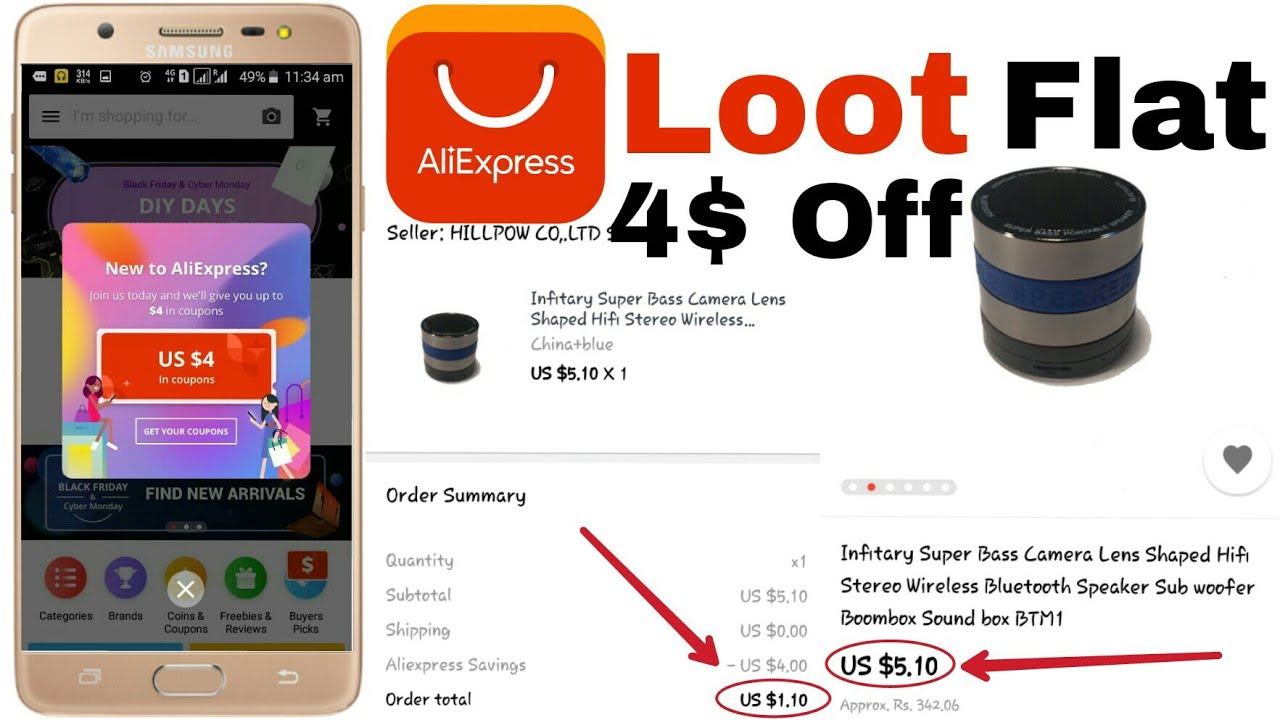The image features a Samsung cell phone prominently displayed on the left-hand side, showcasing its full front view. On the screen of the cell phone, there is a pop-up window with a vibrant background in shades of pink, blue, and yellow. The pop-up window contains text that states "New to AliExpress?" and encourages new users to join by offering up to $4 in coupons. Below this message, there's a distinct button labeled "US $4 in coupons."

To the right of the pop-up window, the AliExpress logo is displayed in a 2D block format. Adjacent to the logo, the text "Loot flat" is visible along with a promotional message indicating "$4 off." 

Within the display, there is a highlighted product from the seller HilpoCO/LTD. The item is described as an Infantry Super Base camera lens-shaped hi-fi stereo wireless device. The product is listed at a price of $5.10. Notably, there are two red arrows on the screen: one pointing to "US $1.10," which might signify a discount or promotional price, and another pointing to "US $5.10," which appears to be the original or listed price of the item.